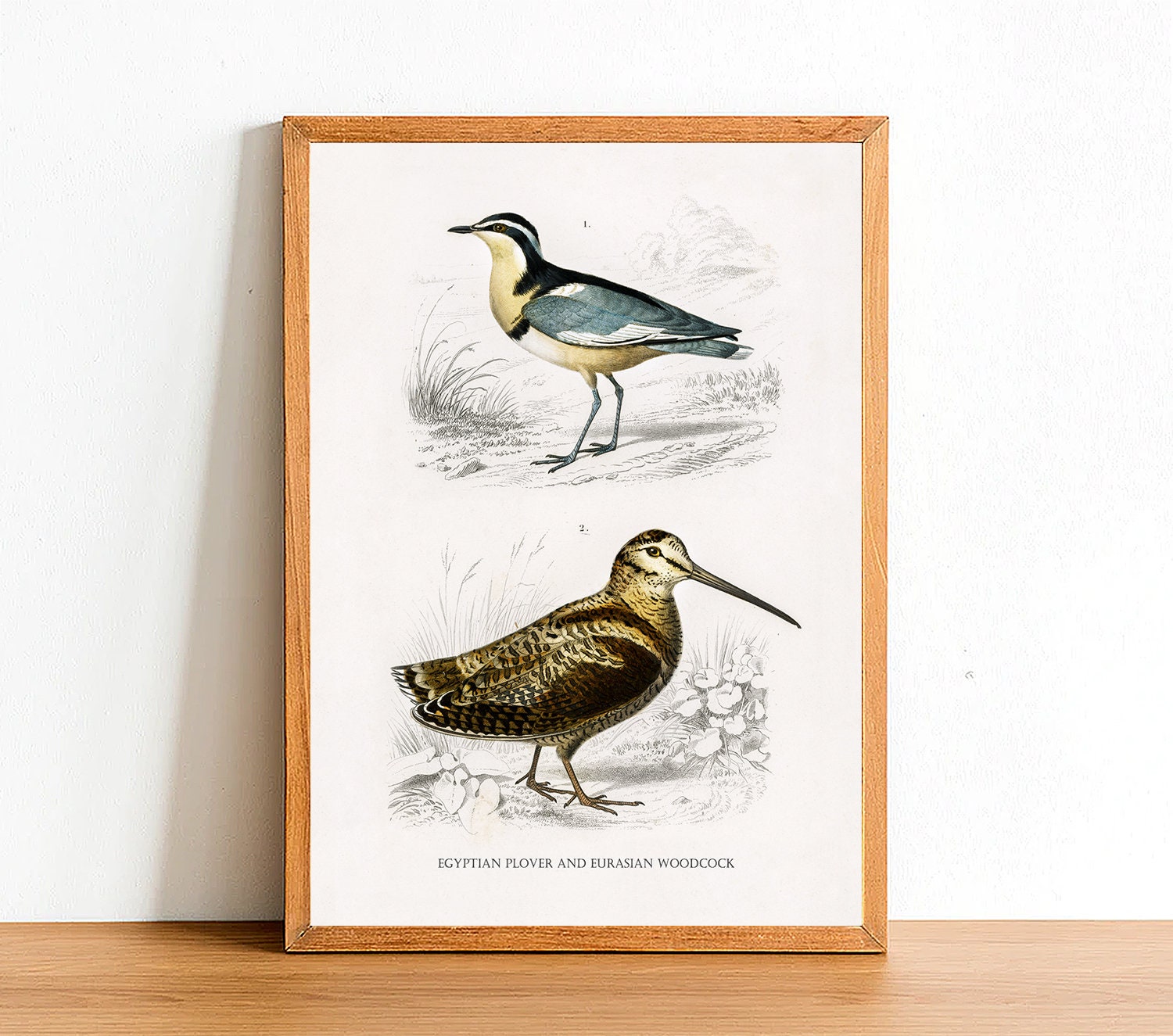This image depicts a detailed artwork of two birds, each labeled as "Egyptian Plover" and "Eurasian Woodcock." The artwork is encased in a light brown wooden frame and sits on a platform with a wooden-like design, leaning against a white wall. There is a visible shadow cast by the frame on the white wall behind it. The platform beneath the artwork is light brown, resembling a wooden table or floor.

The first bird, situated on the top, is facing left. It has a black beak, black eye, and a face adorned with black and white markings. Its neck sports a yellow coloration, while its feathers are a mix of white and light blue. The second bird, positioned below the first, features a long, thin, pointy beak. Its feathers display a blend of brown and tan. This meticulous presentation provides a clear and aesthetically pleasing representation of the two bird species. The text at the bottom of the artwork clearly identifies the birds as an "Egyptian Plover" and an "Eurasian Woodcock."